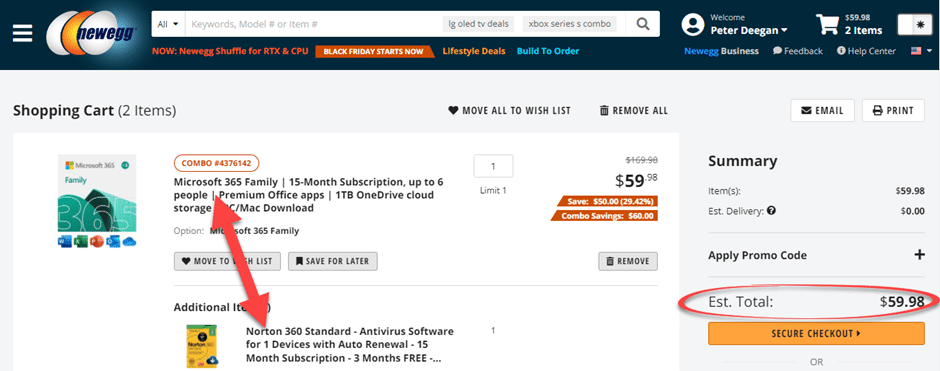In this image taken from the NewEgg website, the top section features the logo consisting of three eggs – a white one, an orange one, and another white one. Overlaying these eggs is the site's name, "newegg," displayed in lowercase, navy-colored letters, all concatenated as a single word: N-E-W-E-G-G. 

Directly beneath the logo, there's a search bar prompting users to input their keyword or model number. In addition, there are highlighted sections for special deals, such as one for TV deals and another advertising an Xbox Series S combo. 

On the right side of the header, the site welcomes the user, Peter Deegan, and indicates that his shopping cart contains two items valued at a total of $59.98. The total amount is notably circled with a red mark for emphasis.

Further down on the right-hand side, the image shows details of a combo deal featuring a Microsoft 365 Family 15-month subscription for up to six people. The package includes premium Office apps and 1TB of OneDrive cloud storage. A red double-ended arrow, indicating importance or a promotion, points up and down over this section.